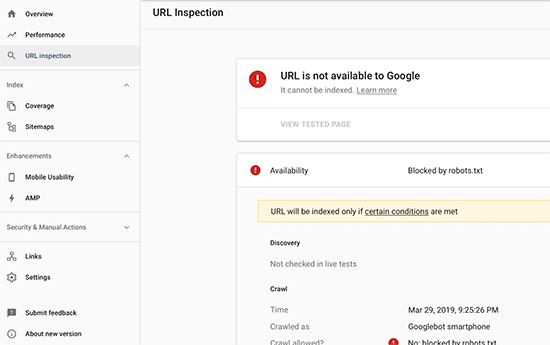**Detailed Descriptive Caption:**

The image is a screenshot of Google Search Console's URL Inspection Tool, displaying crucial details about a particular URL that is not eligible for indexing by Google. The interface is structured with a navigational sidebar on the left featuring multiple sections, including "Main Dashboard Overview," "Analytics on Website Performance," "Indexing Status of Site Pages," "Sitemaps Submitted to Google," "Enhancements," "Mobile Usability," "AMP (Accelerated Mobile Pages)," "Security and Manual Actions" (with subsections for any security issues or manual actions taken by Google), "Links," "Settings," "Submit Feedback," and "About New Versions."

The content area prominently showcases the URL Inspection section with a conspicuous red warning icon, accompanied by the message "URL is not available to Google." This message is further detailed, explaining that the URL cannot be indexed, and it includes a "Learn More" link for additional context. Below the primary warning, there is a "View Tested Page" button for further insights into the issue.

The Availability section reiterates the problem with another red warning icon, stating that the URL is "Blocked by robots.txt," and highlighting that the URL will only be indexed if certain conditions are met, which are linked for reference. It also notes that the URL has "Not Checked in Live Tests."

Further details include the crawl attempt information, which occurred on March 29, 2019, at 9:25:26 PM, carried out by Googlebot Smartphone. The crawl result confirms "Crawled? No, Blocked by robots.txt."

In essence, this interface is meticulously designed to provide in-depth information about the reasons preventing a specific URL from being indexed by Google, along with clear indicators and potential steps to resolve the issue.